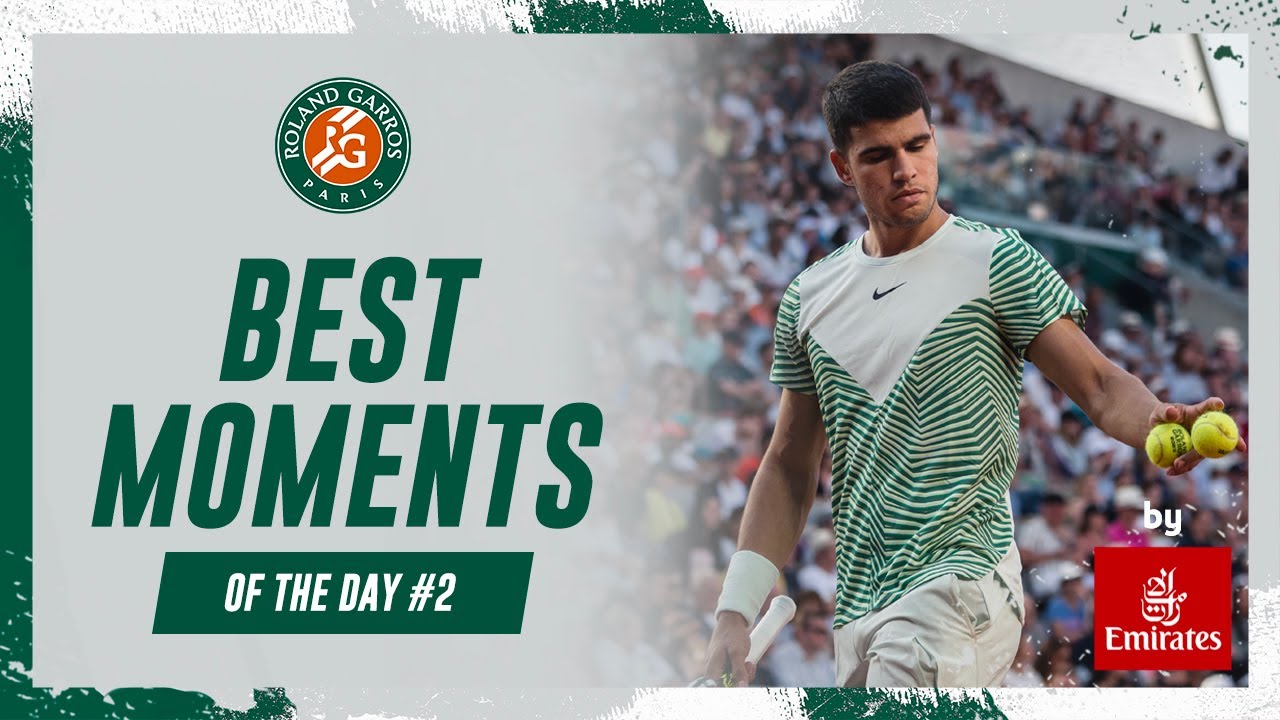The image is a rectangular graphic, measuring approximately five inches wide and three inches high, with a border in green, white, and gray featuring grungy paint strokes. On the left half of the image, a gray background fades towards the right into a photograph occupying the right half. 

In the photograph on the right side, a man with light brown skin is wearing a green-and-off-white striped Nike shirt with a black swoosh on the chest. He holds two tennis balls in his left hand and a tennis racket in his right. Behind him is a crowd seated in stands.

On the gray background of the left side, there is a circular logo at the top. The circle has a green border with white text that reads "Roland Garros Paris," surrounding an inner red-and-white circle with the letters "RG." Below the circle, large green text says "Best Moments," followed by a green bar at the bottom with white text that reads "Of The Day Number Two," forming the phrase "Best Moments Of The Day Number Two."

In the lower right corner of the image, the word "By" is written in white text above a red square containing the Emirates airline logo in white, indicating the feature is sponsored by Emirates.